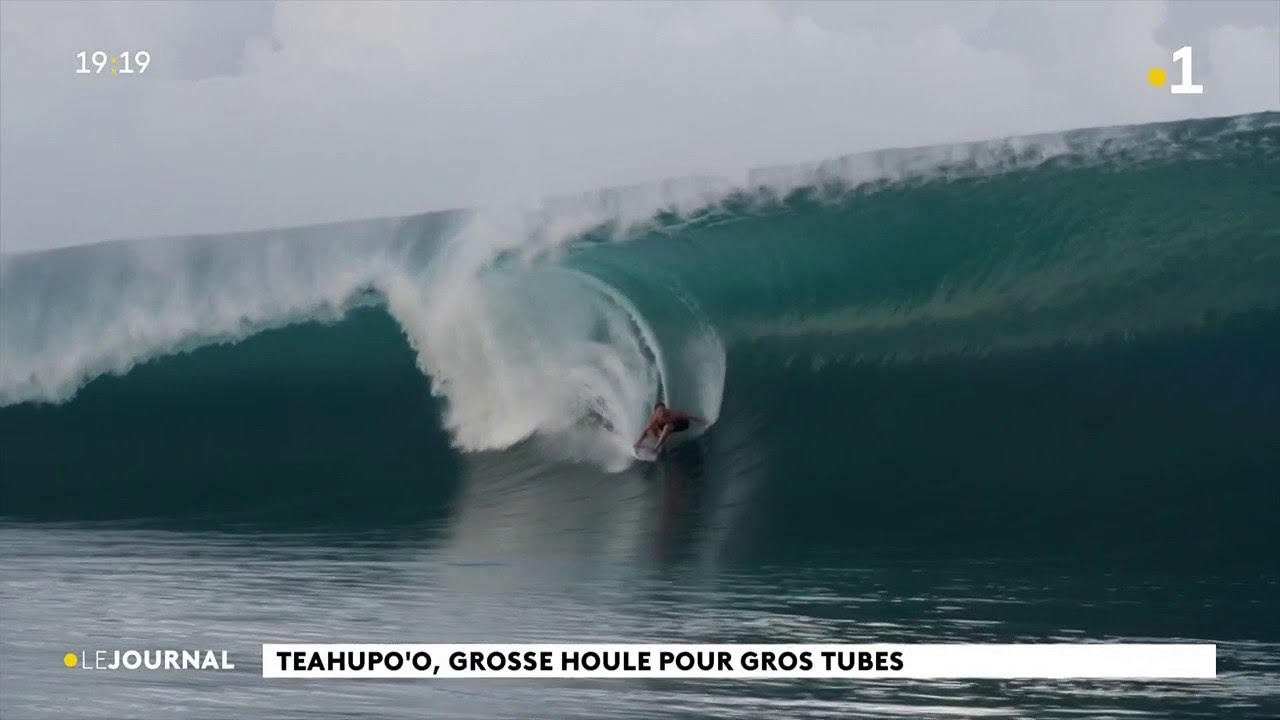The image captures a dramatic moment of a surfer skillfully navigating a massive, curling wave, reminiscent of a liquid tunnel. The giant blue wave, crowned with frothy white foam, looms menacingly behind him, evoking an almost mountainous presence. The surfer is centered in the frame, balancing deftly on his surfboard, one hand gripping the edge to maintain control amidst the dynamic forces of nature. The sky is overcast, adding an element of raw, natural realism to the scene, which is likely framed from a televised broadcast, as indicated by the time "19:19" in the upper left corner and the channel number "1" in the upper right, with a green dot and sun symbol respectively. A headline in French at the bottom left corner, "Le Journal," accompanied by a yellow dot, reads "Tejopo o Grosole por Gros Tubes," further suggesting a report on significant surfing conditions or an event.